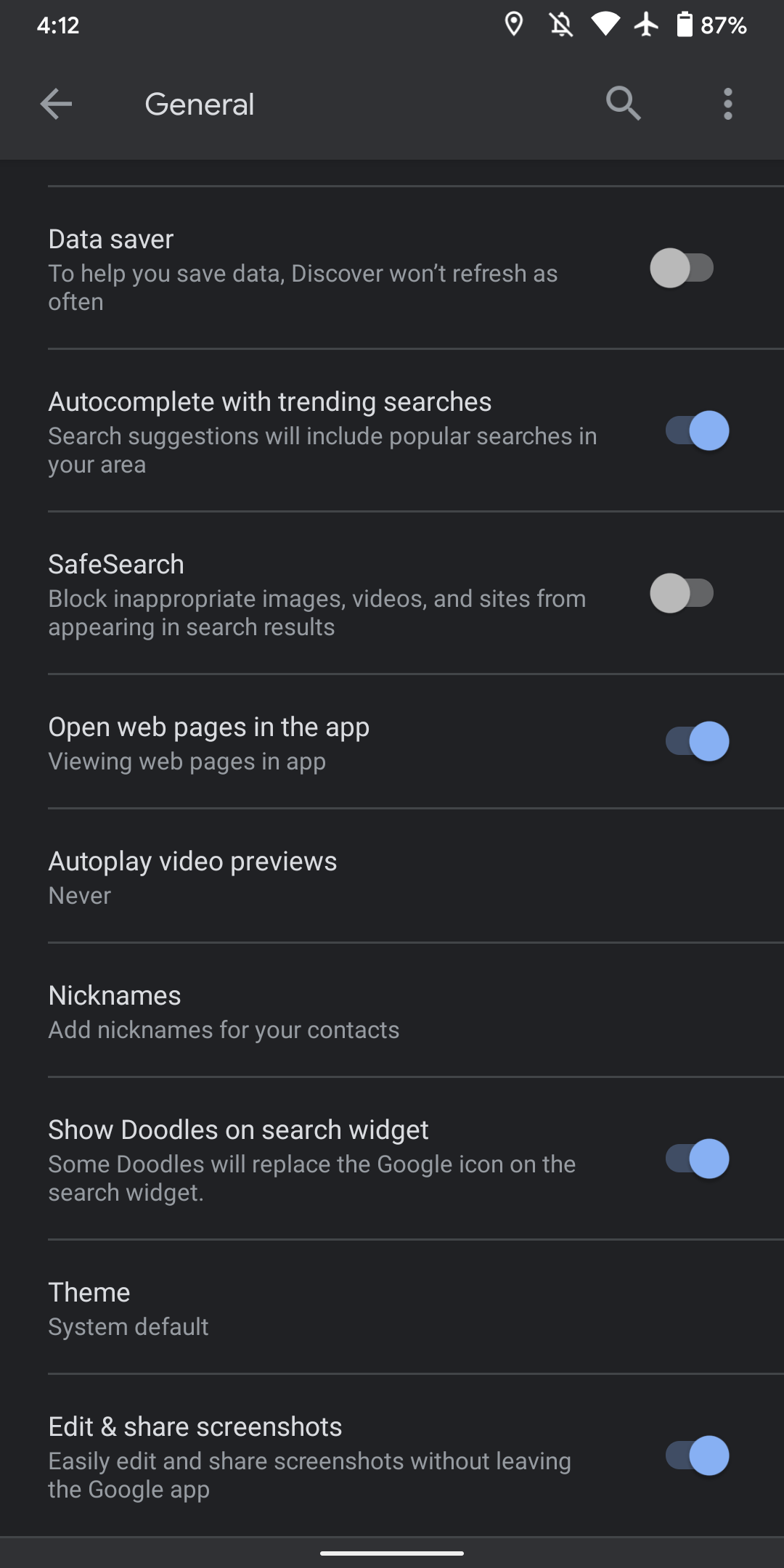A screenshot from a smartphone displays various settings under the "General" tab of an application. In the top left corner, the time reads 4:12. To the right, an array of status icons indicates that the phone is in airplane mode, the alarm is off, the location is on, and the battery is at 87%. 

The "General" heading is positioned beneath a left-pointing arrow, accompanied by a magnifying glass icon, suggesting the presence of a search function.

The settings visible in the screenshot include:

1. **Data Saver**: Helps conserve data by reducing the frequency of Discover refreshes, currently toggled off.
2. **Autocomplete with Trending Searches**: Enables search suggestions that include popular searches in the user's area, toggled on.
3. **SafeSearch**: Blocks inappropriate images, videos, and sites from appearing in search results, toggled off.
4. **Open Web Pages in the App**: Allows web pages to be viewed directly within the app, toggled on.
5. **Autoplay Video Previews**: Set to "Never" for not automatically playing video previews.
6. **Nicknames**: Option to add nicknames for contacts, with no indication of the current status.
7. **Show Doodles on Search Widget**: Replaces the Google icon with themed doodles on the search widget, toggled on.
8. **Theme**: Set to "System Default".
9. **Edit and Share Screenshots**: Allows easy editing and sharing of screenshots without leaving the Google app, toggled on.

The settings options are clearly organized, providing an overview of the app's general configuration at a glance.